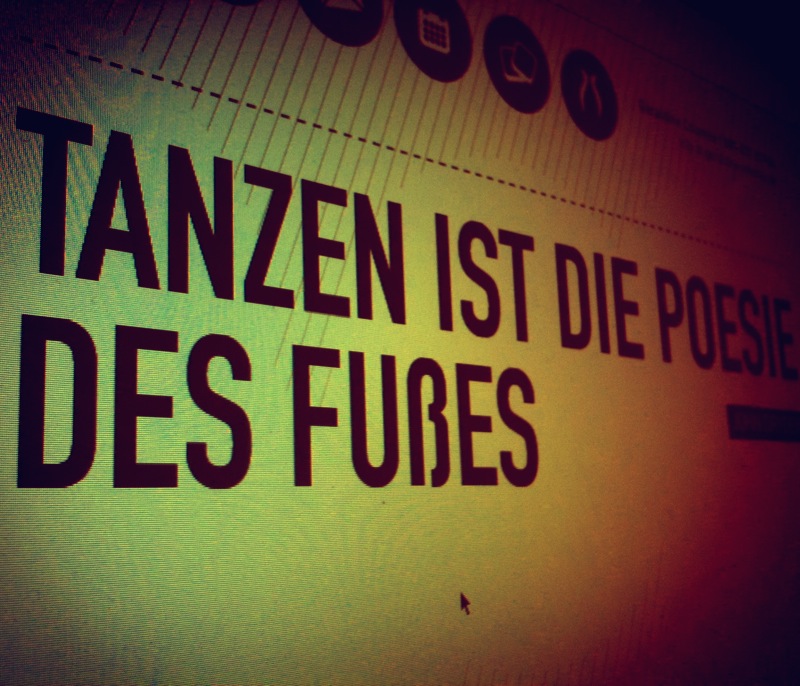This photograph showcases a glowing computer screen prominently featuring the German phrase "Tanzen ist die Poesie des Fußes" in bold black lettering. The background transitions from green at the outer edges to yellow at the center, then shifts to orange and dark red, creating a spotlight effect that adds a vibrant gradient to the image. At the top of the screen, there are four circular icons with indiscernible shapes inside them, separated from the main text by a dotted line. The screen is dark except for this illuminated area, with an arrow cursor visible in the bottom corner, confirming it as a computer interface. Distinct orange slashes and diagonal lines decorate the top part of the screen, enhancing its dynamic appearance.